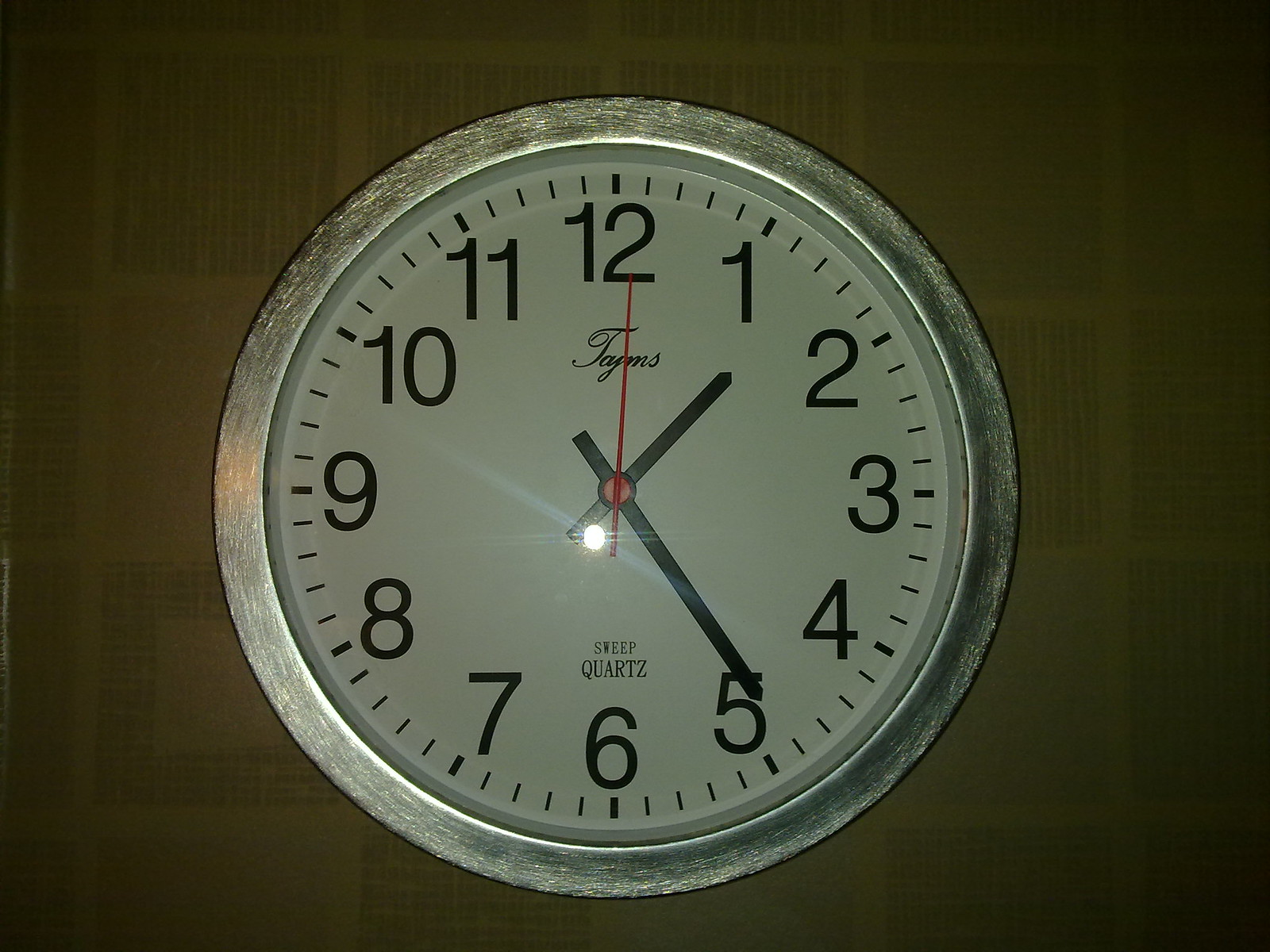The photograph depicts a modern wall clock with a bright and shiny silver rim, highly reflective under the camera's flash. The clock's face is white with standard black Arabic numerals marking each hour from 1 to 12. The hour and minute hands are black, while the second hand is distinctly bright red. Below the 12 o'clock position, in cursive writing, is a brand name that is difficult to decipher. Above the 6 o'clock position, it reads "Steep Courts." The clock indicates the time as 1:24, with the second hand pointing at the 12. The backdrop features a medium brown surface with a grid-like design, somewhat resembling tiles, with darker brown sections inside each square and a faint striped texture. The grid lines are a lighter brown, adding a subtle contrast to the overall pattern.